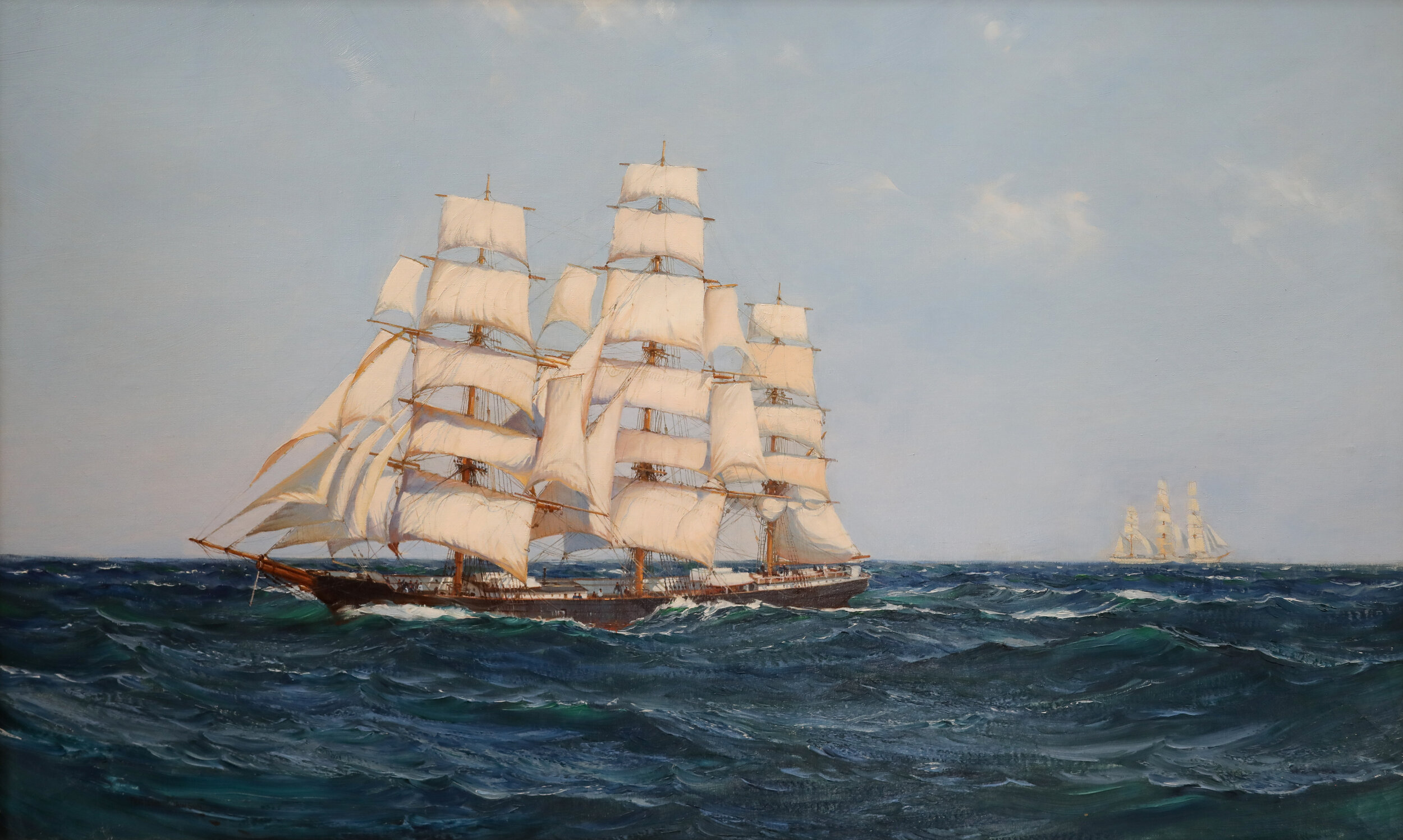The image is a detailed art drawing or painting that showcases a dramatic maritime scene from the Victorian age. It prominently features a massive wooden sailing ship with four towering masts and approximately 20 sails catching the wind. The vessel, seemingly battling through an agitated, dark blue sea with white-capped waves, is navigating towards the left side of the image. The weather above is clear, with a bright blue sky and a few wispy clouds providing a stark contrast to the turbulent waters below. In the background, another large sailboat, also brimming with sails, is sailing in the opposite direction towards the right side of the image, creating a dynamic sense of movement and tension. The distant ship, set against the horizon, adds depth and perspective to this evocative and meticulously detailed maritime artwork.